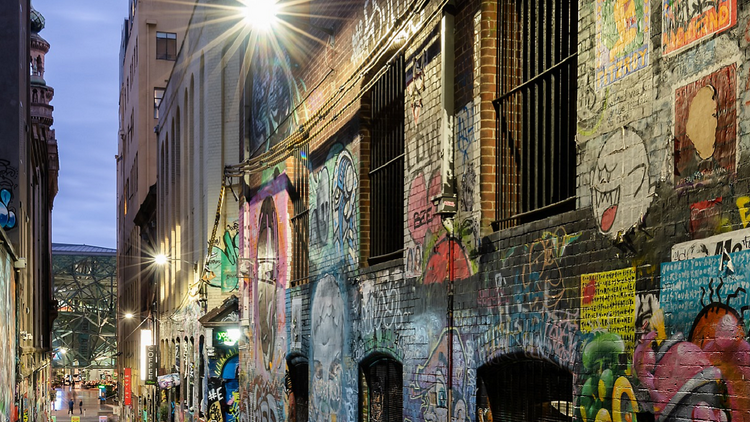This photograph captures an evening scene in a well-lit city alleyway. The tall brick buildings on both sides of the alley are adorned with vibrant graffiti, transforming the space into an open-air art gallery. The graffiti features a wide array of images and text, including a bold man with sharp teeth, a ghost, hearts, the word "love," and brightly colored animals, with prominent hues of purple, pink, green, yellow, red, and white. Several windows of the nearby buildings are barred, adding an urban texture to the scene. At ground level, a few people are seen milling around, possibly shopping, near storefronts that are topped with billboard signs. In the distant background, under the glow of streetlights, a large structure with numerous glass windows—likely a stadium or mall—looms into view, indicating a bustling area beyond the alley. The photograph appears to be taken from a higher vantage point—perhaps the second story—offering a comprehensive view down the alley.